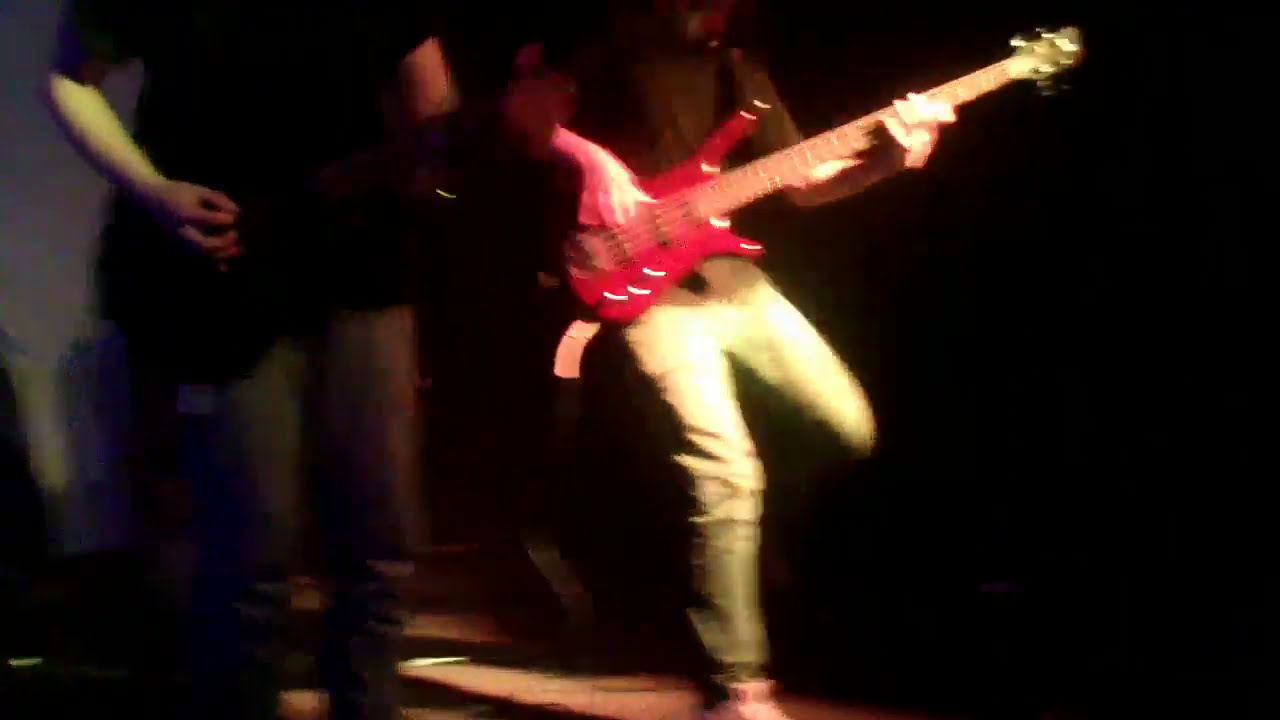In this blurry image, two musicians are captured performing indoors, possibly on a small stage or in a dimly lit room resembling someone's house. Both individuals are positioned centrally on a wooden floor. The scene is predominantly dark, with a black background and minimal lighting, contributing to the overall graininess. The musician on the right, who is kneeling with one foot balancing, is playing a red electric bass guitar. He is dressed in a black t-shirt, gray jeans, and brown boots. To his left stands another musician, wearing a black t-shirt, jeans, and possibly black Converse shoes, playing what appears to be a guitar, although this is obscured by shadows. The darkened lower left part of the image and the lack of visible text or additional objects create a focused yet obscure representation of the performance, highlighting the musicians amidst a backdrop of obscurity.